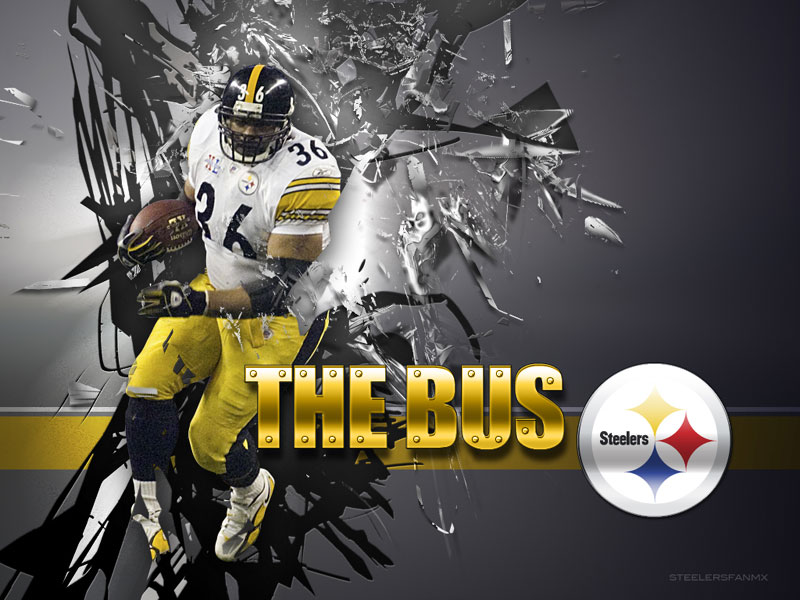The advertisement features a dynamic and striking visual of football player Jerome Bettis, famously known as "The Bus." Set against a gray background that artistically resembles shattering glass on the left side, Bettis appears to be crashing through the image with powerful momentum. He is fully outfitted in his team gear, wearing a black helmet with a yellow stripe, a white and yellow jersey emblazoned with the number 36 on the chest, shoulders, and helmet, and bright yellow pants with a black stripe. His footwear consists of yellow and white cleats. Bettis is depicted holding a brown football in his hands, with his dark brown skin contrasting against his uniform. Prominently displayed in large, bright gold block letters that appear as if they are made of steel and fastened with small screws, the text reads "The Bus." To the right of Bettis is the Pittsburgh Steelers' logo— a white circle featuring yellow, red, and blue stars, accompanied by the word "Steelers" in black text. A subtle yellow stripe runs horizontally across the bottom of the image, adding a cohesive touch to the overall design. The detailed and high-energy composition captures the essence of both Bettis's prowess and the Steelers' brand.